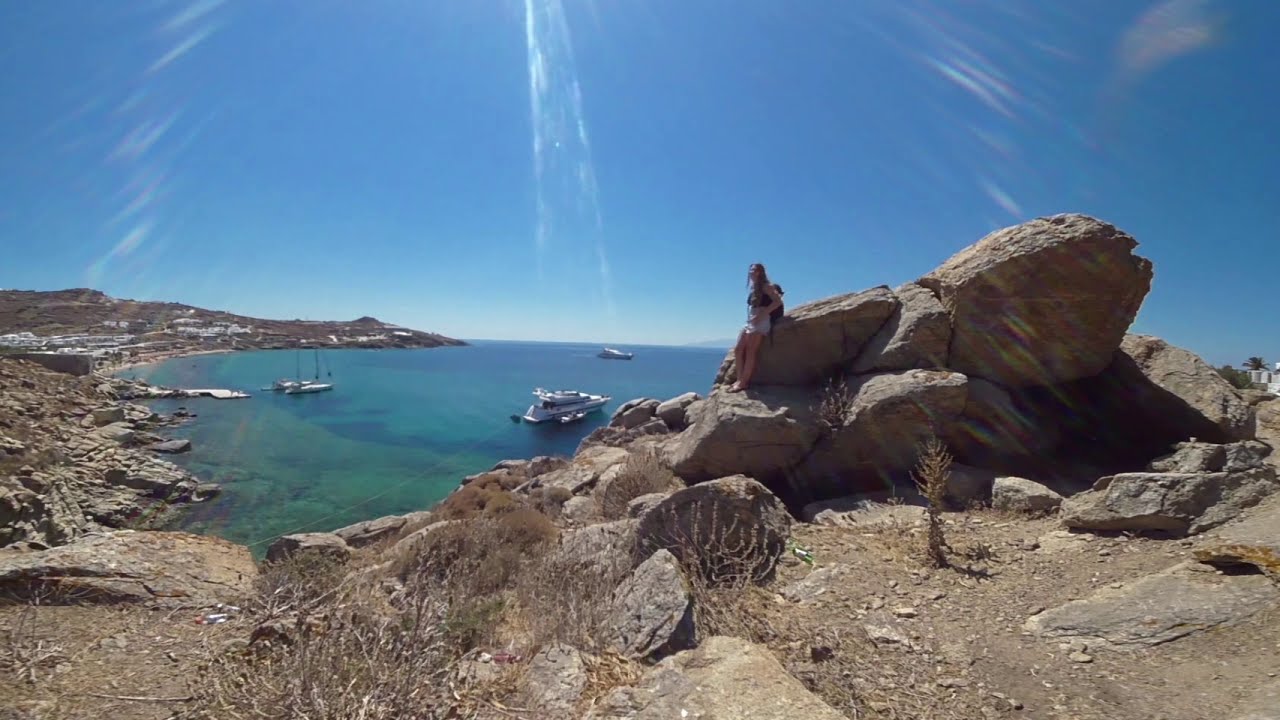In this vibrant photograph taken on a bright, sunny day in a tropical area, the upper half showcases a brilliant blue sky with striking bursts of sunbeams cascading down, reminiscent of a Star Trek teleportation scene. On the bottom half, the scenery reveals a rugged, rocky landscape interspersed with sparse, desert-like vegetation. Dominating the right side, a Caucasian woman with white shorts, a black top, and a black backpack leans against a large rock formation. The rocky terrain continues around an oval cliffside to the left, barren but dotted with what appear to be dead or dried desert plants.

In the background, the clear, greenish-blue waters contrast beautifully against the rocky shore. The water closest to the shore is greenish-blue, giving way to deeper blue hues towards the horizon. At least three yachts float on the serene water, accompanied by a distant cruise ship possibly heading towards a small dock on the far left. Near the dock, a few white buildings stand out, hinting at nearby civilization. To the far right, a distant building can be barely discerned amidst the clear day. No other people or animals are visible in this idyllic and tranquil scene.